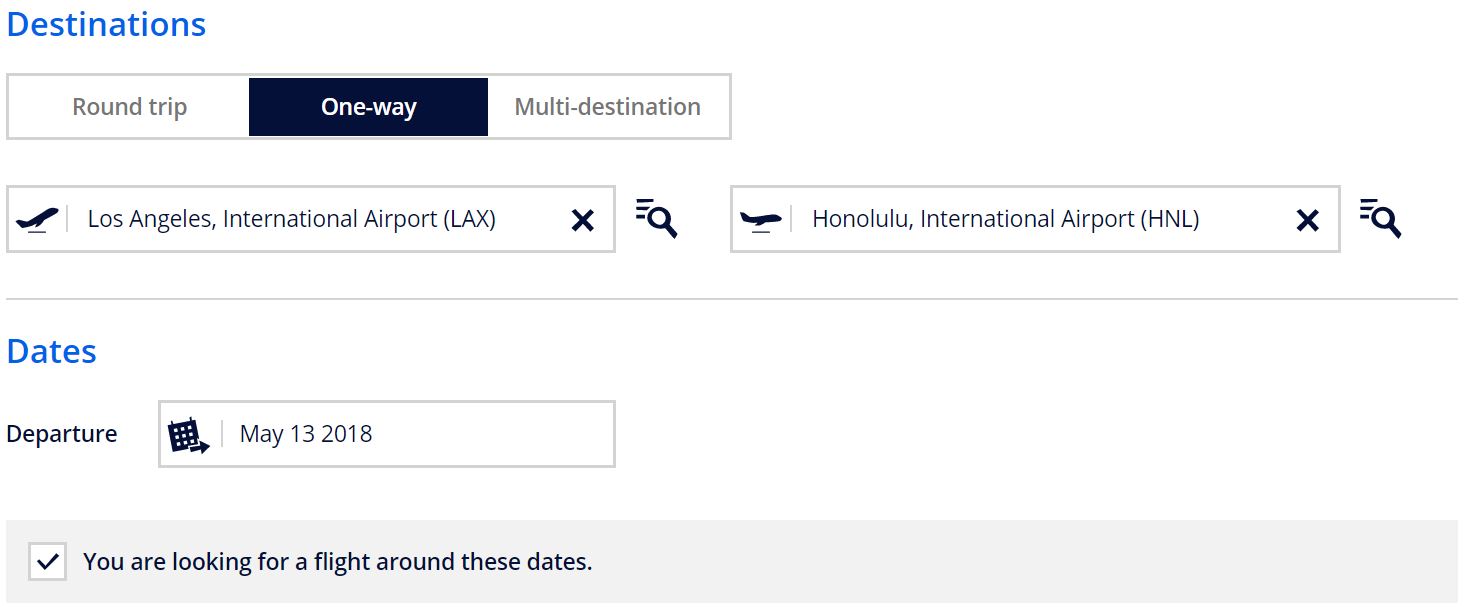The image showcases a flight booking page with a clean and organized layout. 

- **Top Left Corner**: The word "Destination" is prominently displayed in blue, establishing the page's focus on flight bookings.
- **Trip Type Section**: Beneath the destination header, three trip options are presented - "Round-Trip," "One-Way," and "Multi-Destination." The selected option, "One-Way," stands out with a dark blue background, contrasting the white background and black text of the other two options.
- **Flight Details**:
  - **Departure**: The journey starts from Los Angeles International Airport (LAX).
  - **Arrival**: The destination is Honolulu International Airport (HNL).
  - A "Clear" button is available for resetting entered information.

- **Date Section**: 
  - Located below the departure details, the word "Date" is highlighted in blue.
  - The selected departure date is May 13, 2018.
  - A checked checkbox indicates the user is interested in flights around this date. This checkbox is featured on a light gray background, adding subtle emphasis.

- **Background**: The main background color of the page remains white, offering a clean and minimalistic look, with the dark blue trip type selection providing a striking visual contrast.